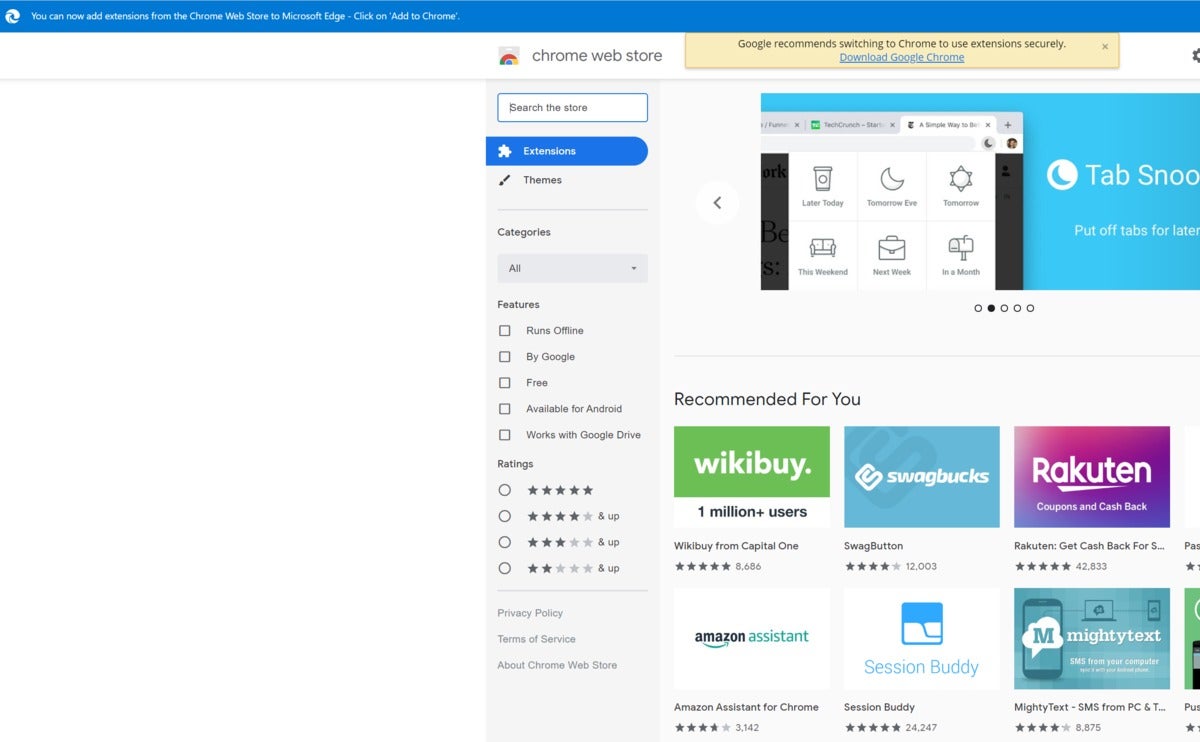This image captures the Google Chrome Web Store's main interface. At the very top, a blue bar features the Google Chrome logo in white on the left corner. Adjacent to this, white text announces, "You can now add extensions from the Chrome Web Store to Microsoft Edge. Click on add to Chrome."

Beneath the blue bar, there is a white bar showcasing the Google Chrome Web Store logo. Centered at the top, bold text urges users that "Google recommends switching to Chrome to use extensions securely. Download Google Chrome." To the left of this message is the search store box, accompanied by tabs like extensions, themes, categories, features, ratings, and links to the privacy policy, terms of service, and other information about the Chrome Web Store.

On the right side, a tab cycles through various apps. In the lower right section of the image, there is a "Recommended for you" section displaying several add-ons such as Capital One's Eno, SwagButton, Rakuten, Amazon Assistant for Chrome, Session Buddy, and MightyText SMS from PC.